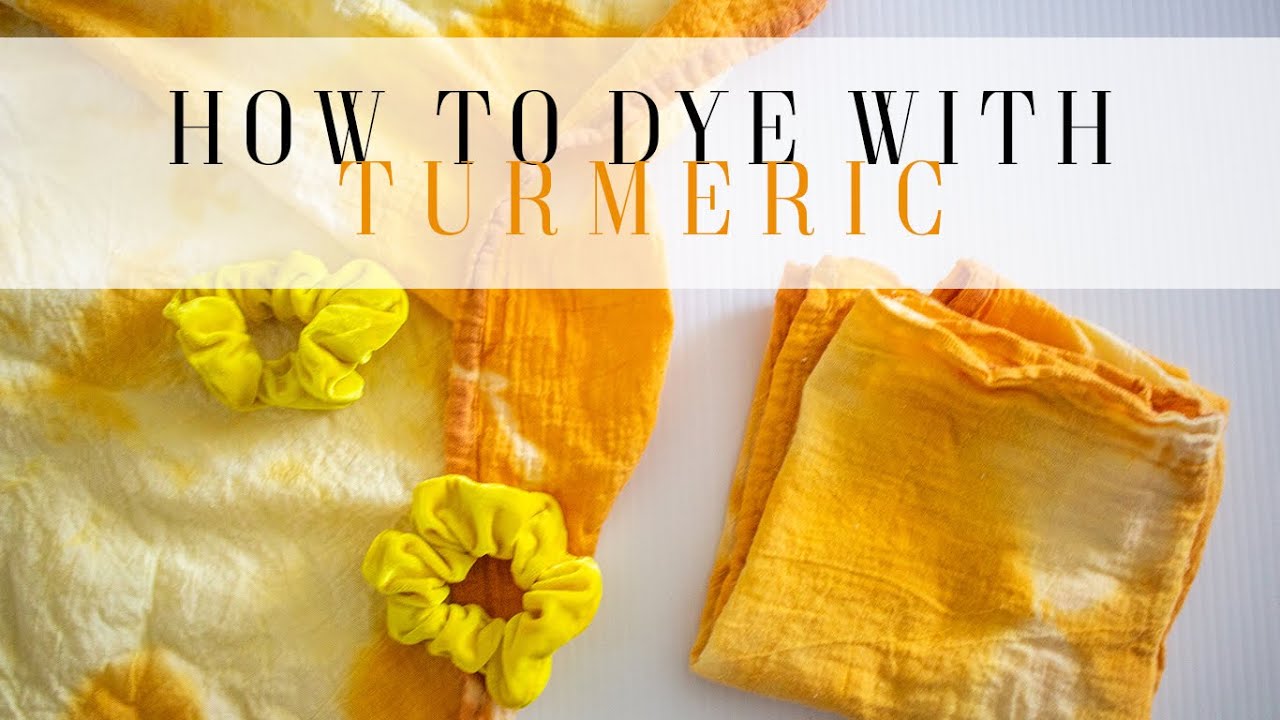This photograph serves as an illustrative guide on using turmeric as a natural fabric dye. It features a translucent white bar overlay at the top with the title "How to Dye with Turmeric" printed in black and dark orange font, reminiscent of turmeric’s vibrant color. On a white background, possibly a table, there are two distinct cloth pieces: one folded into squares showcasing an orange and cream tie-dye pattern, and the other laid out flat with similar coloration. Accompanying these fabrics are two yellow hair scrunchies, positioned one above the other on the left side, also likely dyed with turmeric. The overall palette of the image is dominated by shades of white, bright turmeric orange, and yellow, creating a cohesive visual representation of the dyeing process.